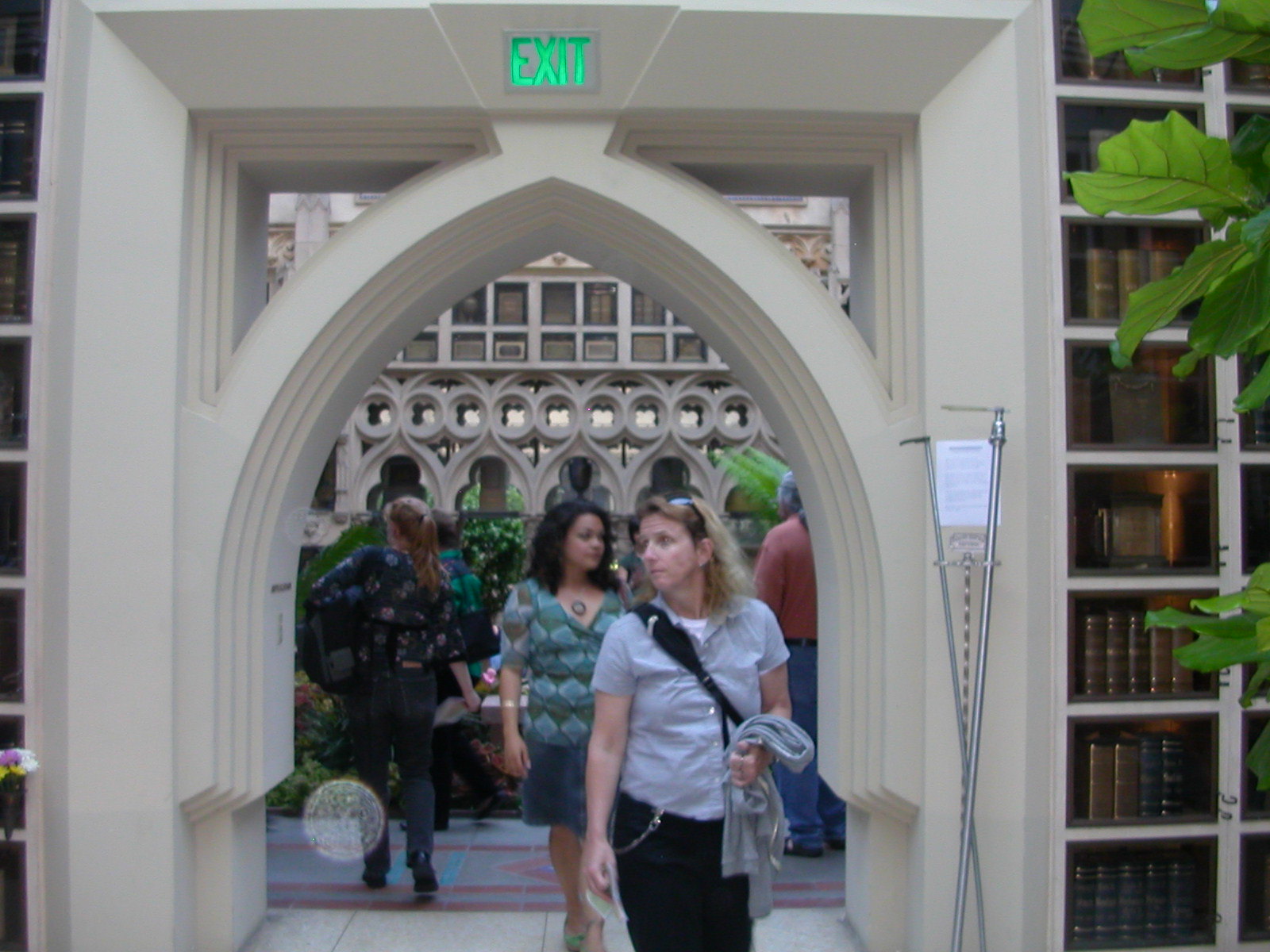In this detailed photograph, two women are captured walking through a large, light-colored stone archway that serves as an entrance and exit to a building. This arched doorway, resembling the top half of an oval, has no physical door but is crowned by a prominently lit green exit sign at the top center. The interior foreground of the image reveals bookshelves laden with books, possibly suggesting this could be a library. The ornate carved structure or wall is visible in the background beyond the archway, implying a blend of indoor and outdoor environments accentuated by visible greenery and outdoor plants.

The woman leading the way through the archway sports blonde hair, held back by sunglasses. She is dressed in a light blue top and dark pants adorned with a chain at the belt, and she's carrying a sweater over her shoulder. Following her is another woman with shoulder-length dark hair, wearing a denim skirt paired with a blue printed top and a large statement necklace.

On the right side of the image, apart from the bookshelves, there appears to be a pole forming an X and additional outdoor plants peeking through, consolidating the image's rich, detailed setting.